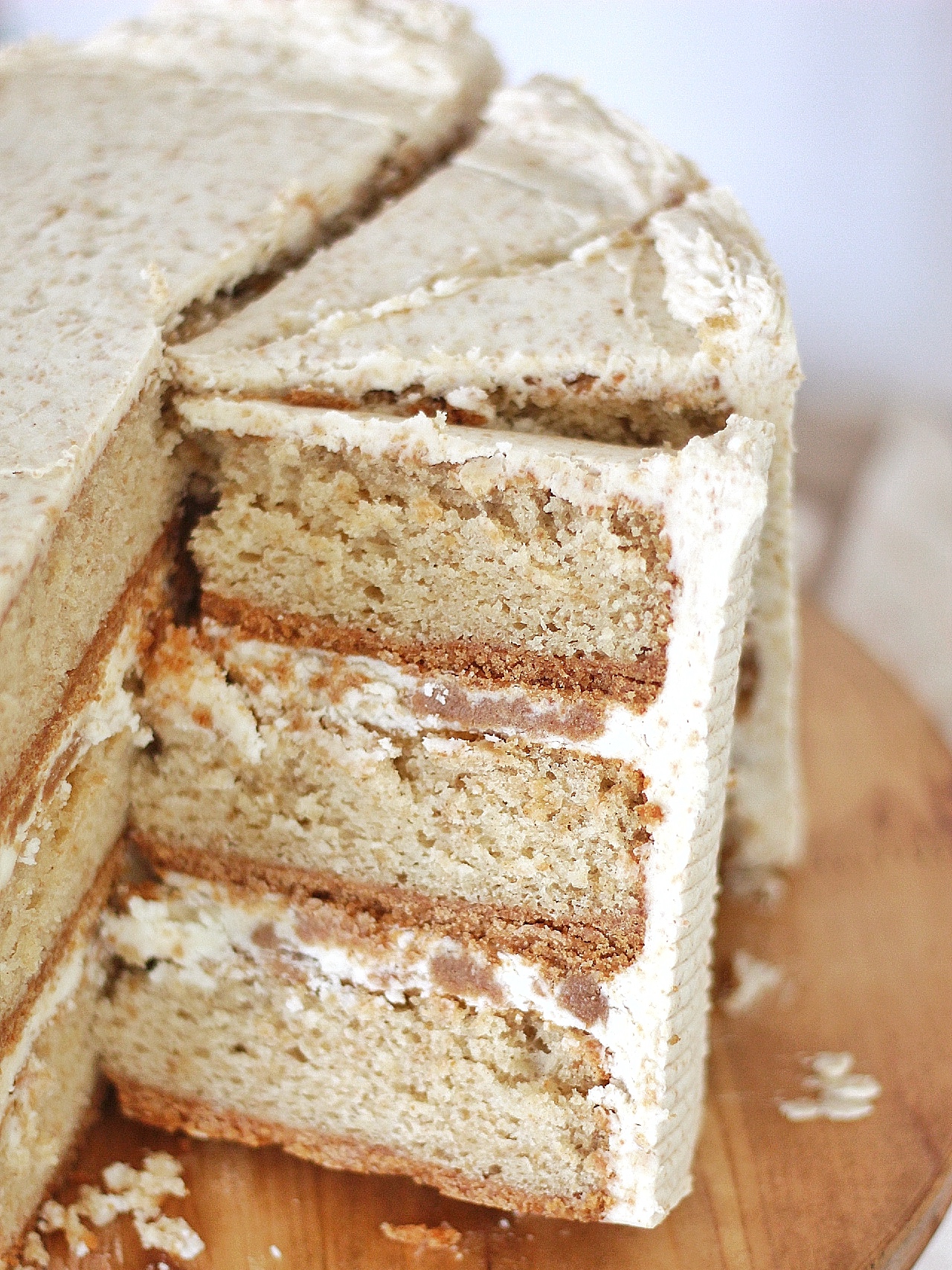This image showcases a close-up, color photograph of a delectable three-layer cake that has been sliced to reveal its intricate layers. The cake, which appears to be a light tan or light brown color, is displayed on a wooden board or cake platform, with crumbs scattered around. Each layer of the cake is separated by a whitish buttercream frosting speckled with pale brown flecks, adding to its visual appeal and suggesting a rich, moist texture perhaps enhanced by a syrup. The same frosting is also artfully applied over the top and down the sides of the cake. Only about half of the circular cake is visible due to the close-up nature of the photo, emphasizing the cross-section and its detailed layers. The cake features a decorative buttercream border on top, and three slices have been cut out, making it an enticing subject for a cookbook or food photography.